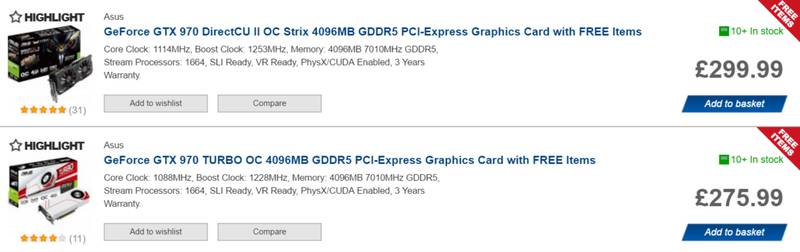The image showcases a section of a shopping website with a clean, white background, focusing on two product listings side by side.

### First Listing (Left-hand Side):
- **Logo**: Top left corner, a black-outlined star with a white center and the word "HIGHLIGHT" in all capital letters.
- **Product Image**: Displayed in front of a box.
- **Rating**: Five yellow stars and the text "31 reviews" in parentheses.
- **Product Name**: "ASUS GeForce GTX 970 DirectCU II OC Strix 4096 MB GDDR5 PCI Express Graphics Card with Free Items"
- **Specifications**: 
  - Core Clock: 1114 MHz
  - Boost Clock: 1253 MHz
  - Memory: 4096 MB, 7010 MHz GDDR5
  - Stream Processors: 1664
  - SLI Ready, VR Ready, PhysX-CUDA enabled
  - Warranty: 3 years
- **Actions**:
  - Gray button with black text: "Add to Wishlist"
  - Gray button with black text: "Compare"
- **Additional Information**:
  - Red triangle in the upper right corner with white text: "Free Items"
  - Stock Information: "10+ in stock" in gray text
  - **Price**: £299.99
  - Blue button with white text: "Add to Basket"

### Second Listing (Right-hand Side):
- **Logo**: Features the same black-outlined star with a white center and the word "HIGHLIGHT" in all capital letters.
- **Product Image**: Displayed in front of the box.
- **Rating**: Four yellow stars and the text "11 reviews" in parentheses.
- **Product Name**: "ASUS GeForce GTX 970 Turbo OC 4096 MB GDDR5 PCI Express Graphics Card with Free Items"
- **Specifications**:
  - Core Clock: 1088 MHz
  - Boost Clock: 1228 MHz
  - Memory: 4096 MB, 7010 MHz GDDR5
  - Stream Processors: 1664
  - SLI Ready, VR Ready, PhysX-CUDA enabled
  - Warranty: 3 years
- **Actions**:
  - Gray button with black text: "Add to Wishlist"
  - Gray button with black text: "Compare"
- **Additional Information**:
  - Red triangle in the upper-right corner with white text: "Free Items"
  - Stock Information: "10+ in stock" in gray text
  - **Price**: £275.99
  - Blue button with white text: "Add to Basket"

Both products highlight key specifications, reviews, stock availability, and interactive buttons to enhance the shopping experience.